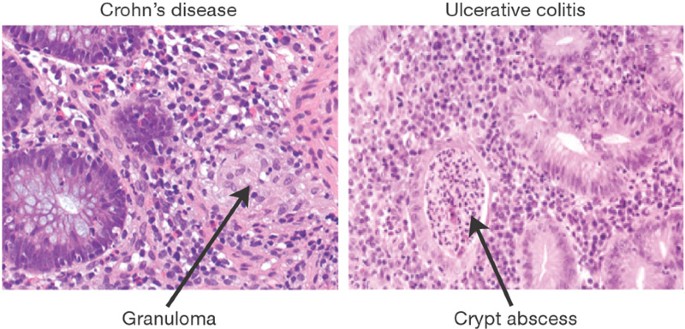The image consists of two side-by-side microscopic photos of cells, each depicting a different medical condition. Both images are set against a plain white background and separated by a thin vertical white bar. Each photo features a distinct label at the top and another identifier at the bottom, with corresponding black arrows indicating specific areas.

The left image is labeled "Crohn's Disease" at the top. Below, it displays a granular cell pattern in varying shades of purple and lavender, interspersed with dark purple dots and small white spaces. At the bottom, the label "Granuloma" is prominently displayed, with a black arrow pointing to a specific region characterized by light pink swirls and a darkish pink spot.

The right image is labeled "Ulcerative Colitis" at the top. This image has a more uniform appearance, showcasing a light purple and white background filled with consistently distributed purple dots. The bottom of the image features the label "Crypt Abscess," with a black arrow pointing to a highlighted area that is marked by a ring of light pink surrounding dense pink and purple dots, including a highlighted white region.

The overall design and labeling of the images aim to highlight and compare the distinct cellular differences between Crohn's Disease and Ulcerative Colitis.